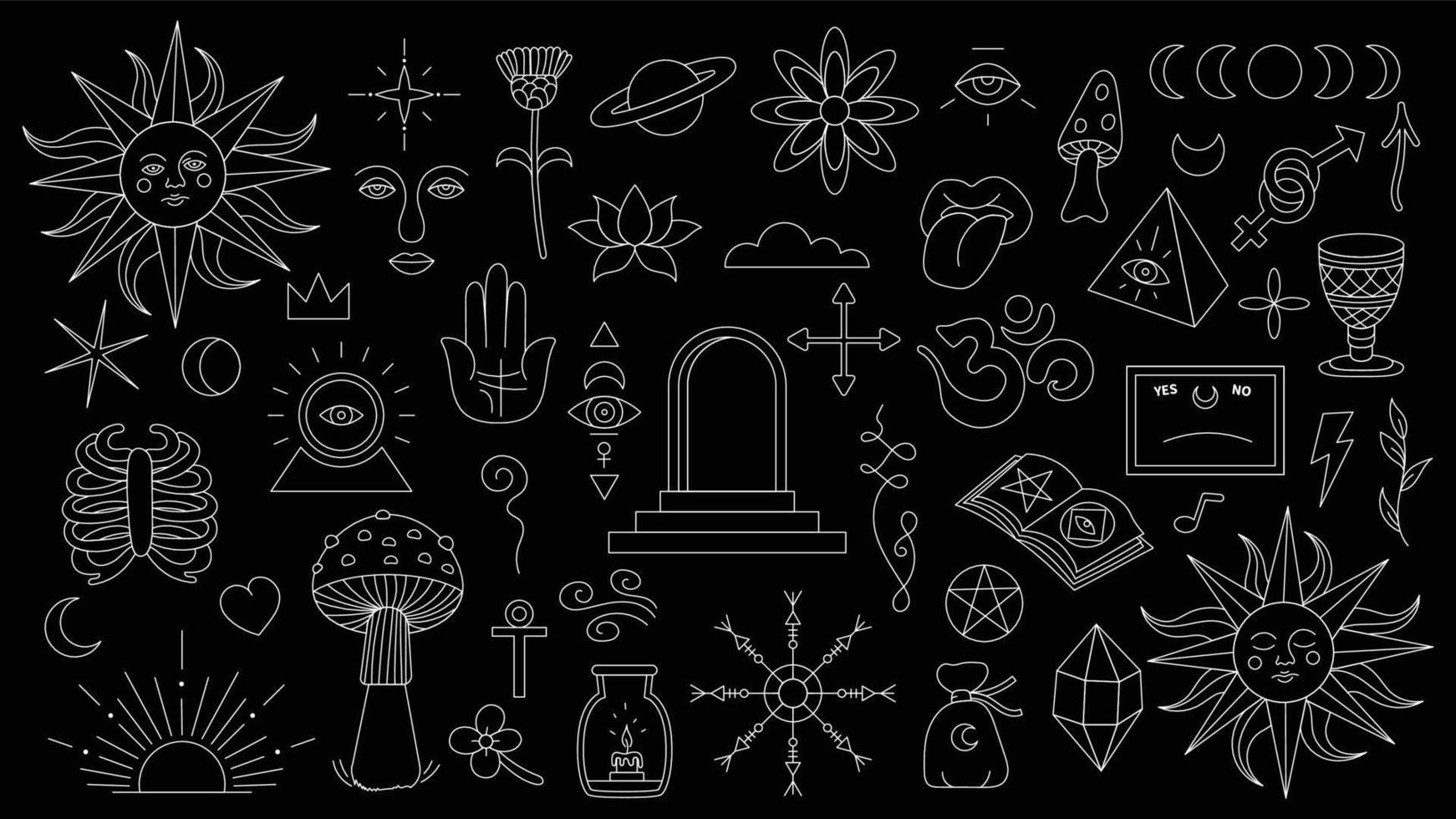On a large, black, horizontally oriented rectangle, an array of intricate, white, outline doodles cover every inch, creating a chaotic yet fascinating visual narrative reminiscent of chalk drawings on a chalkboard. The upper left corner is dominated by a sun with a face, radiating wavy and straight pointy rays, while an adjacent northern star keeps it company. Multiple suns with faces, including one with closed eyes, are scattered across the image, contributing to its celestial theme.

Various elements evoking a sense of mysticism and the occult are distributed throughout the design. Notable symbols include a pyramid with an all-seeing eye, a mouth with a tongue sticking out—a symbol often associated with the all-mocking tongue—a lotus flower, a rib cage, and a hamsa hand. Intertwined male and female symbols point to the theme of unity, while the OM symbol invokes a spiritual undertone.

Additionally, there are numerous astrological and cosmic references: planets with rings, crescent moons, and the different phases of the moon. Terrestrial and fantastical elements coexist, such as mushrooms, chalices, and lightning bolts. A compass, an arched doorway with steps, and a music note introduce elements of navigation and creativity.

Further enriching the composition are objects like a candle in a face, a clover, a diamond, a crown, and a bag with a rope tied around it. Books—one open with a five-pointed star and another possibly related to occult texts—emphasize the esoteric nature of the collage. There are multiple, repetitive symbols like the all-seeing eye and clouds, contributing to the overall busy yet enthralling atmosphere of the image.